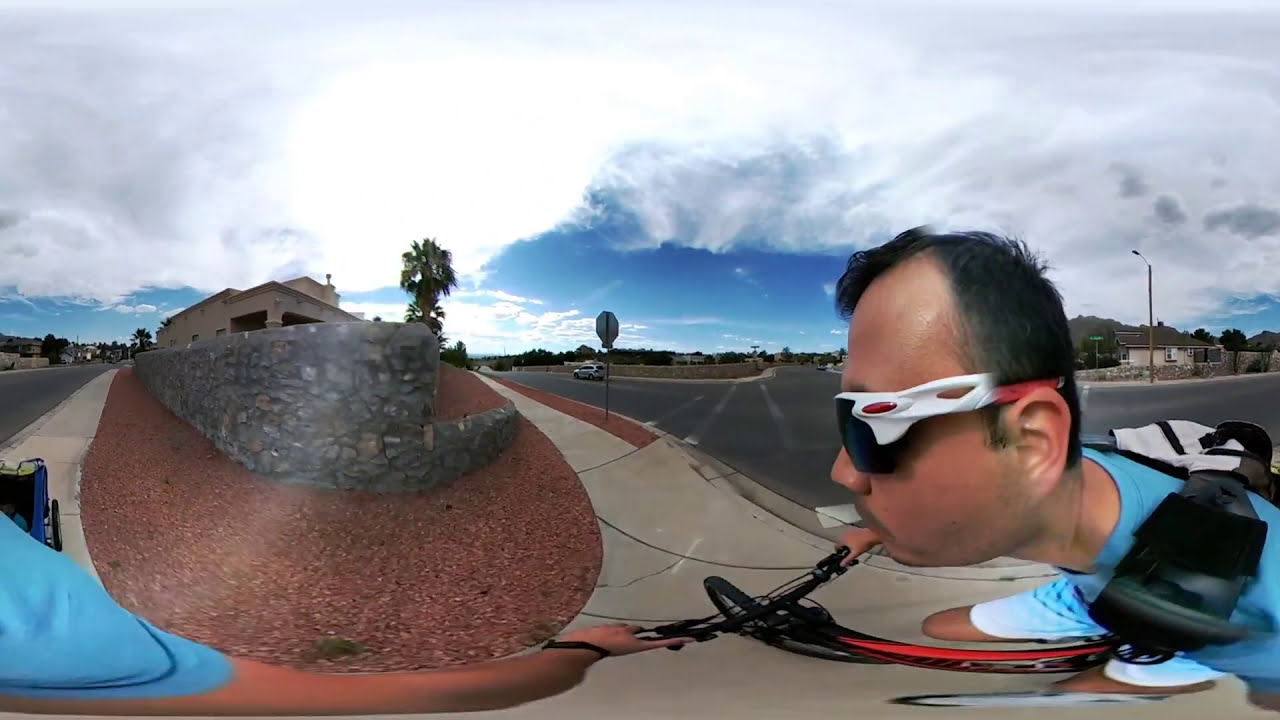The photograph showcases a fisheye-lens image of a man riding a black and red mountain bike on a sidewalk in a residential area. The lens distortion warps the scene, making it appear as though the camera is mounted near the man's elbow, offering a wide-angle perspective. The man has short dark hair and is wearing white sunglasses with red accents, a turquoise blue t-shirt, and matching turquoise blue shorts. He also has a backpack on. The sky above him is a bright blue with partial cloud coverage, suggesting an overcast day with the sun attempting to shine through. The background reveals a residential neighborhood featuring a freshly paved black road, a stone wall with some red rock and a stone building with a triangular roof on the left. Palm trees and a gray sidewalk further detail the surroundings. The complex warping of the image gives a unique, almost distorted, view of the scene, making details like a close-up of the pavement appear as an unusual round shape in the photograph.